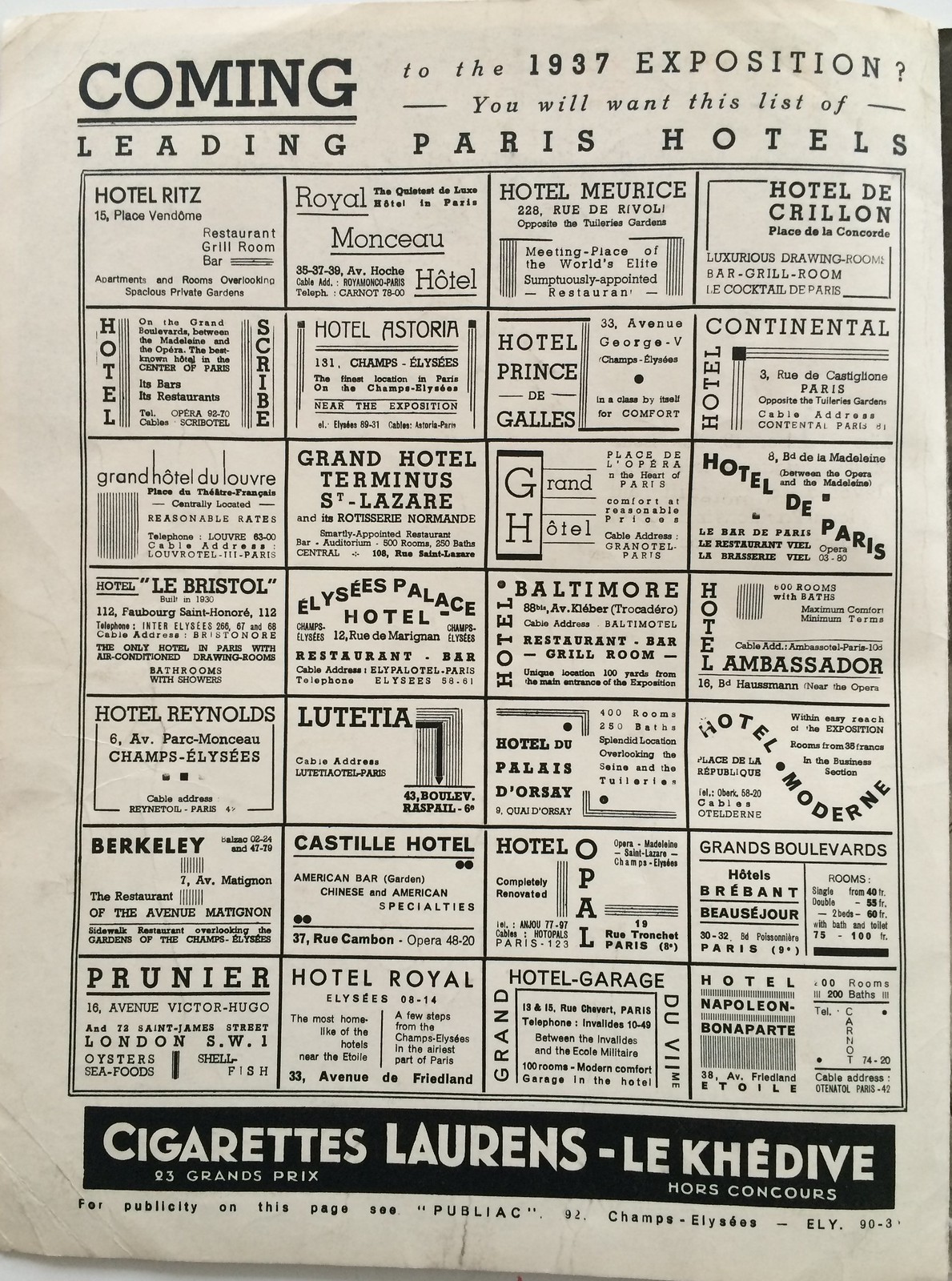This image is a black-and-white photograph of a page from an old magazine or booklet, featuring advertisements primarily for Paris hotels in anticipation of the 1937 Exposition. The page is white with black lettering. At the top, it prominently states: "Coming to the 1937 Exposition? You will want this list of leading Paris hotels." Below this header, a grid of advertisements for various hotels is displayed in a four-by-six arrangement. Some notable listings include the Hotel Ritz at 15 Place Vendôme, featuring amenities like a restaurant, grill, room, bar, and apartments with garden views, the Royal Monceau Hotel, and Hotel Astoria located at 131 Champs-Élysées, touted as having the finest location near the exposition. Below these hotel advertisements, there is an ad that reads "Cigarettes Laurens des Cadavres, 93 Grand Prix, Ours Concours," and at the very bottom of the page, small print notes: "For publicity on this page, C. Publiac, 92 Champs-Elysées."